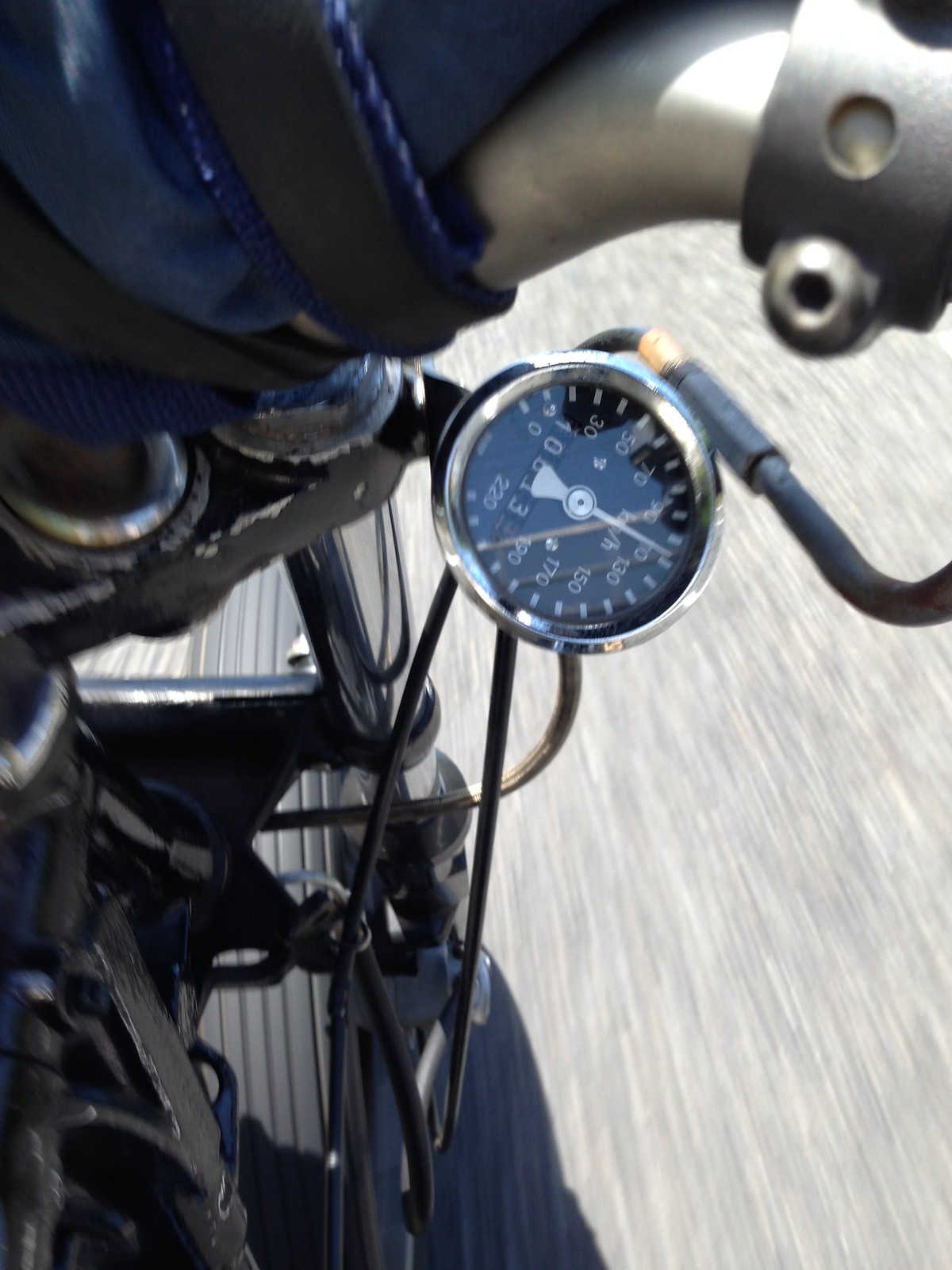A dynamic first-person perspective captures the thrilling experience of riding a motorcycle at high speed. The camera, positioned on the right side of the bike and pointed downwards, reveals the blurred motion of the asphalt rushing by. The front tire is visible with motion lines that emphasize the bike's swift pace. Attached to the right handlebar, a wire trails back into the motorcycle's inner workings, connecting to a kilometers-per-hour speedometer that indicates a speed of approximately 98 to 100 km/h. Partially visible in the bottom left is the black frame of the bike, including the right suspension pole connected to the tire frame and rim. In the top left corner, blue clothing with black straps appears, hinting that the rider’s hand, perhaps equipped with a camera, captures this exhilarating moment mid-ride. The clear asphalt and the sleek design of the motorcycle suggest this is a high-performance road bike.